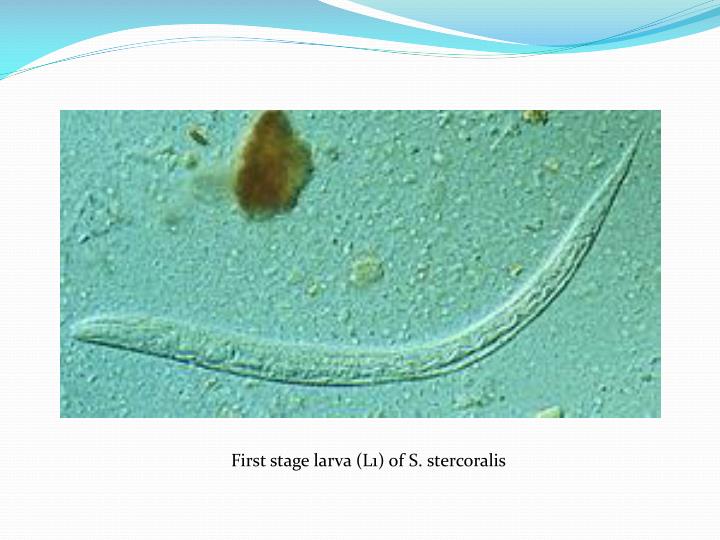The image features a rectangular layout, approximately 6 inches wide by 5 inches tall, with a smaller inset photograph about 2 inches tall by 4 inches wide. The image background consists of a light tannish blue hue, topped with a sky blue border featuring waves.

The photograph within this layout depicts a turquoise, underwater-like scene observed through a microscope, showing intricate grains and particles. The primary focus is a snake-like or worm-like organism that stretches from the lower left corner to the upper right corner, with a pointed tail. Surrounding the organism are various bumps and blobs in shades of aqua, light brown, and dark brown, with the most prominent blob being dark brown and located near the top just left of center.

Below the photograph, black text on a white background reads: "First Stage Larvae (L1) of S. stercoralis."